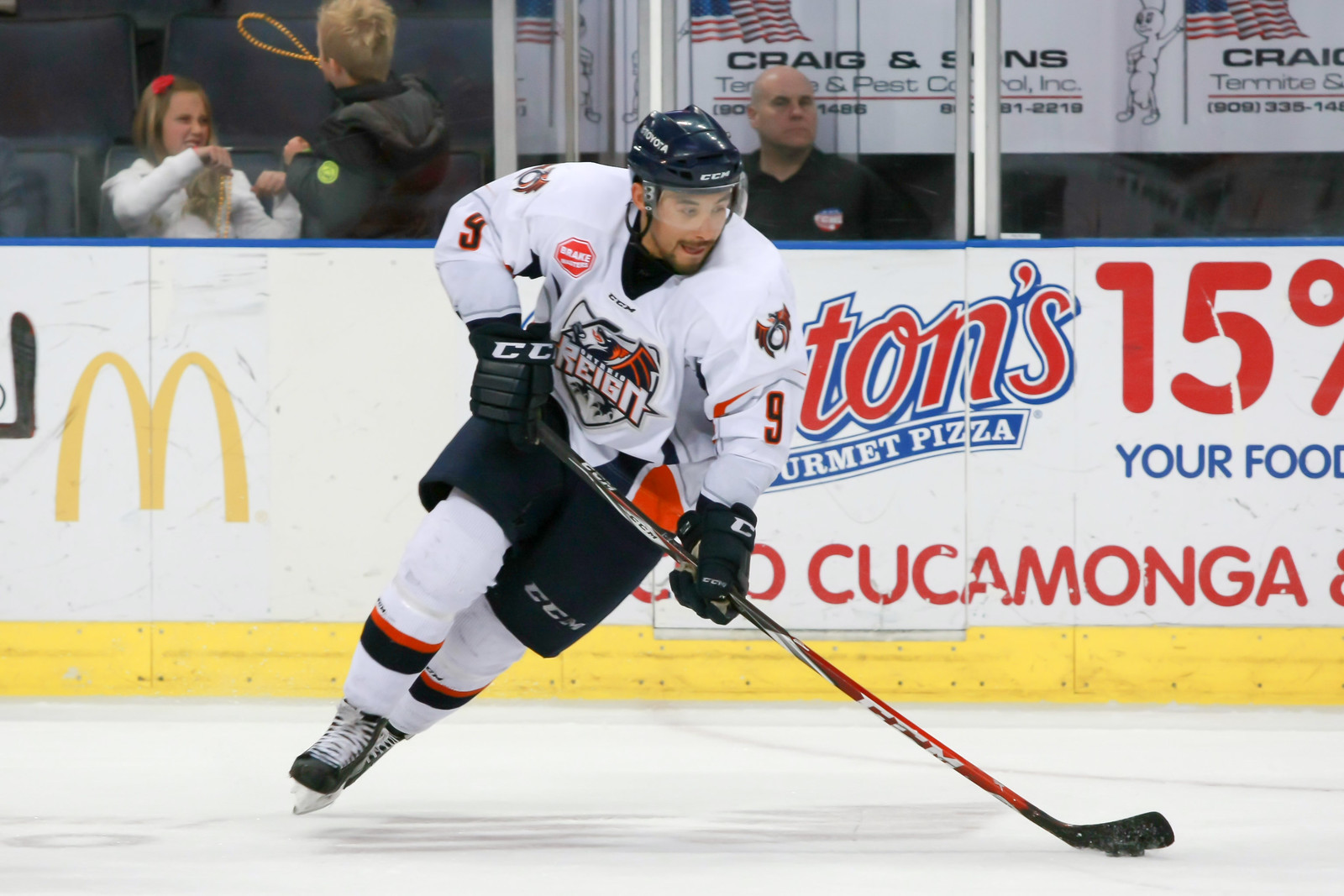In the image, there is a male ice hockey player with a mustache and goatee at the center of the action. He is on the ice in a rink and poised with his black and white hockey stick, lining up to hit a puck. The player is dressed in a complete team uniform, consisting of a white jersey with the word "REIGN" emblazoned on a seal pattern on his chest, as well as the number ‘line’ displayed on both arms. He sports a blue helmet, black shorts, pads, gloves, and skates. His stance is slightly slanted, with his focus directed to the right side of the image.

The ice rink itself is surrounded by advertisement boards, displaying sponsors such as McDonald's, Stunz Gourmet Pizza, Cucamonga, and others. In the audience area behind these boards, to the left of the player, sits a woman and a child engaging with each other, suggesting they are watching the game. Further to the right, another bald-headed man in a black shirt is attentively watching the match. The white ice and boundary walls set a stark contrast, with flags and additional banners, such as one labeled "Kray-Gensunz" bearing a U.S. flag, reinforcing the atmosphere of an exciting live game.